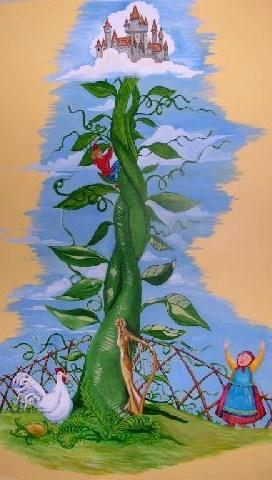The illustration depicts a classic scene from Jack and the Beanstalk, portrayed within a tall, vertical rectangle with a tan background. The scene is set against a backdrop of a blue sky with irregularly edged clouds. Dominating the center is a colossal green beanstalk, which starts off pale green at the bottom and intensifies in color as it ascends. The beanstalk is bursting from the ground, breaking through a supporting fence, and is adorned with giant leaves and tendrils.

Ascending the beanstalk about two-thirds of the way up is Jack, easily identifiable by his red shirt and blue pants, with yellow hair peeking out. At the very top of the beanstalk, perched amidst the clouds, is a grand gray and red castle with multiple turrets.

At the base of the beanstalk, there is a white chicken, seemingly having just laid an egg, likely golden. Nearby, a farm woman, presumed to be Jack’s mother, is positioned at the bottom right. She is dressed in a red dress with yellow sleeves, a blue apron, and has her head wrapped in a handkerchief. Her arms are raised, gazing intently up at Jack as he climbs, though her exact emotions are ambiguous.

The illustration captures the fantastical ascent from the ground up to the castle in the clouds, with every detail contributing to the classic tale’s magical and adventurous atmosphere.